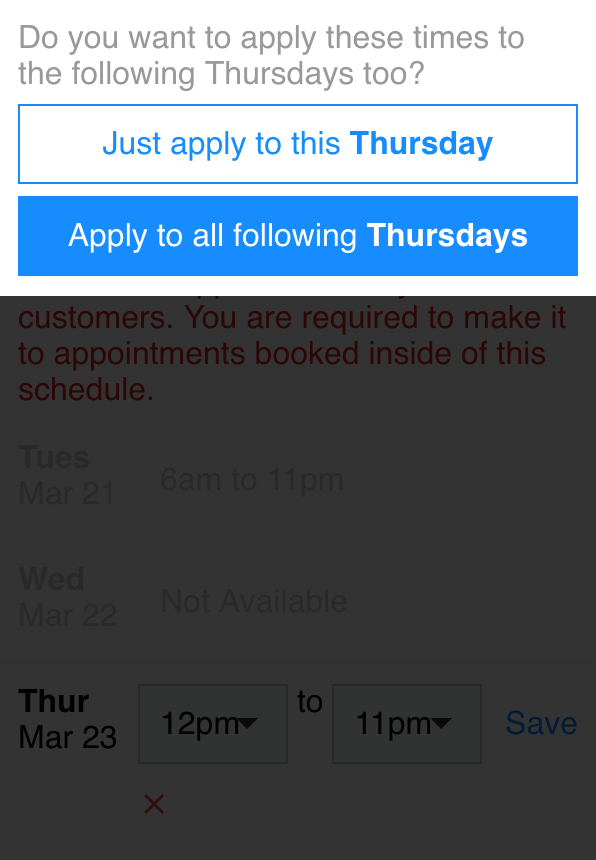The image portrays a user interface with a white background at the top featuring a prompt in gray text: "Do you want to apply these times to the following Thursdays too?" Below the prompt are two buttons. The first button is white with a blue font and outline, displaying the text: "Just apply to this Thursday." The second button is blue with white font, reading: "Apply to all following Thursdays." 

The lower section of the interface displays a portion of a website obscured by a gray overlay. Within this section, a red warning message states: "Customers, you are required to make it to appointments booked inside this schedule." 

Following the warning are specific scheduling details: 
- Tuesday, March 21st, 6 a.m. to 11 p.m.
- Wednesday, March 22nd, not available.
- Thursday, March 23rd, 12 p.m. to 11 p.m.

The time slots for Thursday, March 23rd, are presented with dropdown menus, indicating they are currently being adjusted. On the right side of the interface, a "Save" button is visible, associated with the Thursday scheduling adjustments.

The context of the appointments being booked is not specified, nor is the nature of the device being used (whether a cell phone, tablet, or computer). Additionally, there is no indication of the website or application in use, as no URL or branding is visible. The primary action being queried is whether the adjusted times should apply to just the current Thursday or to all following Thursdays.